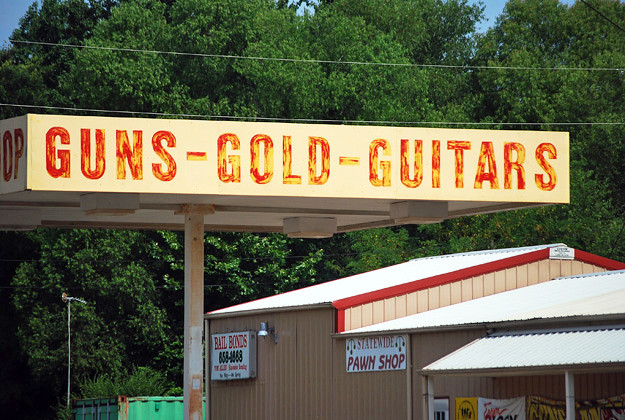The image, captured in vibrant color, features a distinctly Southern American scene. The photograph is horizontally oriented, with the longer side of the rectangle running horizontally. Dominating the backdrop is a building prominently marked with the text "Statewide Pawn Shop" and "Bail Bonds" on its side. The main focal point of the photo is a roof structure reminiscent of a gas station awning, although no fuel pumps are visible beneath it. Bold, capitalized red letters stretch across the roof, spelling out "GUNS - GOLD - GUITARS," with each word separated by a hyphen. The setting sun casts a warm glow, adding to the quintessential Southern atmosphere of the scene.